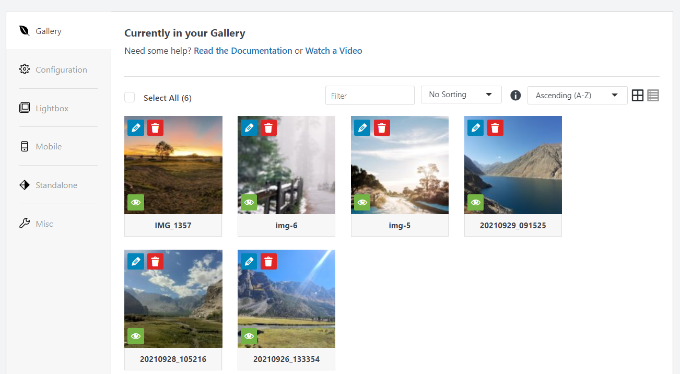A webpage displays a gallery monitor interface. It features a navigation menu on the left-hand side with various icons, including a gallery leaf, a configuration icon, a lightbox labeled "Lightbox," a mobile phone icon for mobile settings, a standalone diamond icon, and a wrench for miscellaneous settings. The gallery section contains instructions to seek help through documentation or video tutorials if needed.

The gallery comprises six photographs arranged in a grid layout: four on the top row and two on the bottom row. Users can select all six images, apply filters, sort them ascending from A to Z, and choose grid viewing options.

Each image in the gallery has a blue edit button at the top, a red delete button, and a green button at the lower left, possibly for HTML code. The images are as follows:

1. **First Image (image_1357):** An outdoor shot of a field at sunset.
2. **Second Image (IMG-6):** A snowy field with trees, a fence, and possibly a road.
3. **Third Image (IMG-5):** Another snowy scene of a road on a bright day.
4. **Fourth Image (20210929_091525):** A mountain lake with barren mountains rising from the water.
5. **Fifth Image (20210928_105216):** A scenic mountain area with a sunny sky and scattered clouds.
6. **Sixth Image (20210926_133354):** A light-filled lake scene dominated by mountains in the background.

The images are labeled with identifiers beneath them for easy reference.